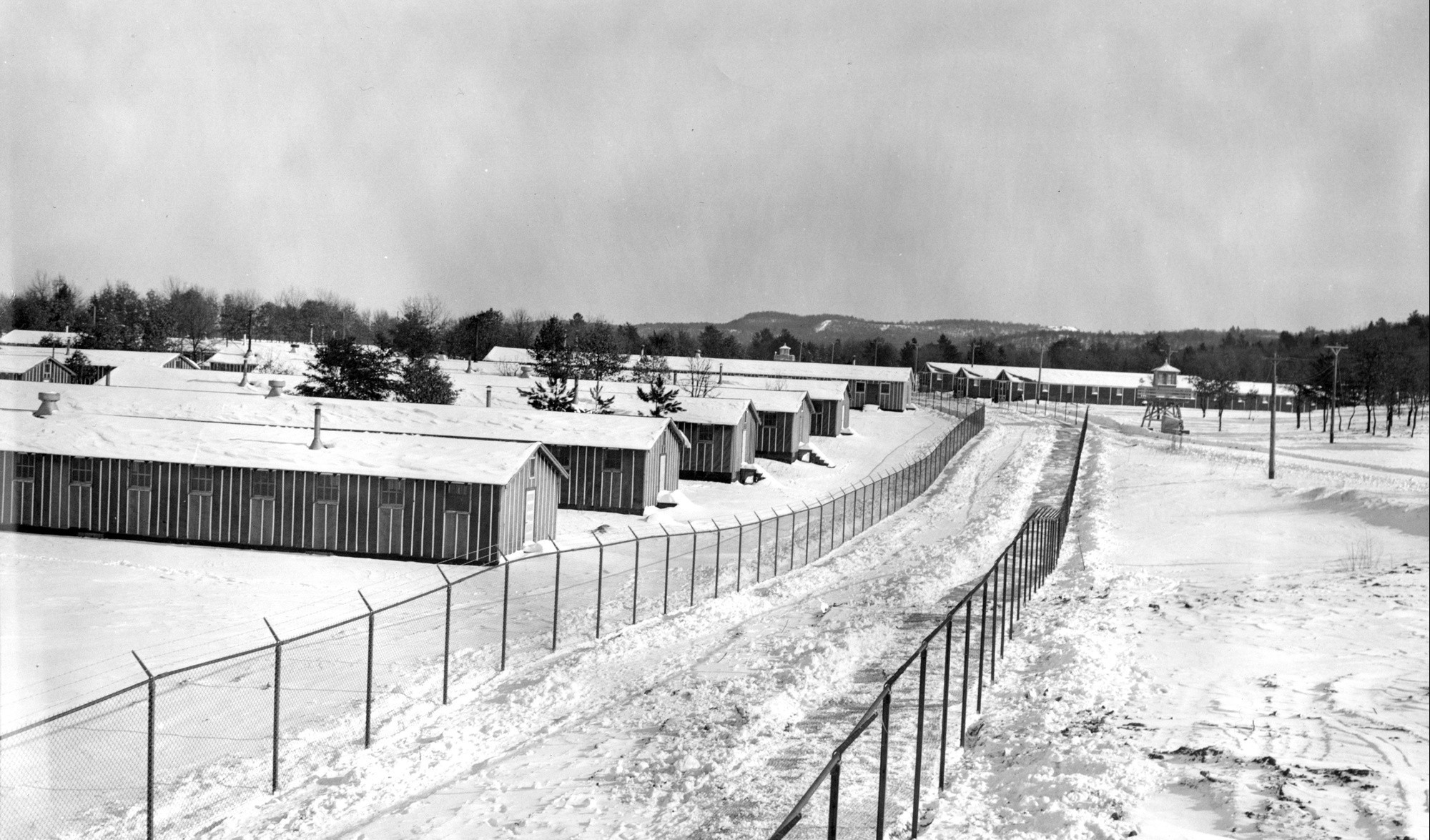The black-and-white photograph captures a vast, snowy landscape reminiscent of a secluded camp, possibly resembling a World War II internment or prison camp in a desolate, Siberia-like environment. The scene is set during the daytime, as indicated by the daylight illuminating the area despite a cloudy sky. Long, narrow buildings line both sides of a walkable or motorable pathway that runs from the bottom left corner toward the horizon, narrowing into the distance. These buildings, resembling dormitories or warehouses, feature multiple small windows, a single door with a window above it, chimneys, and vertical exterior boards. They are uniformly spaced and flanked by a chain-link fence on either side, creating a sense of order and confinement.

Surrounding the camp is a dense forest that stretches up to a range of dark-gray hills or mountains in the background. The stark, icy landscape extends across the entire photograph, covering the ground, rooftops, and trees. Scattered among the buildings are electric poles with wires, suggesting some level of infrastructure. Notably, a rooftop viewing point or overhead tank is visible, along with a prominent watchtower or lookout structure positioned in front of the secondary set of similar buildings on the horizon. The overall scene evokes a cold, isolated, and regimented atmosphere, captured through the lens of vintage black-and-white photography.